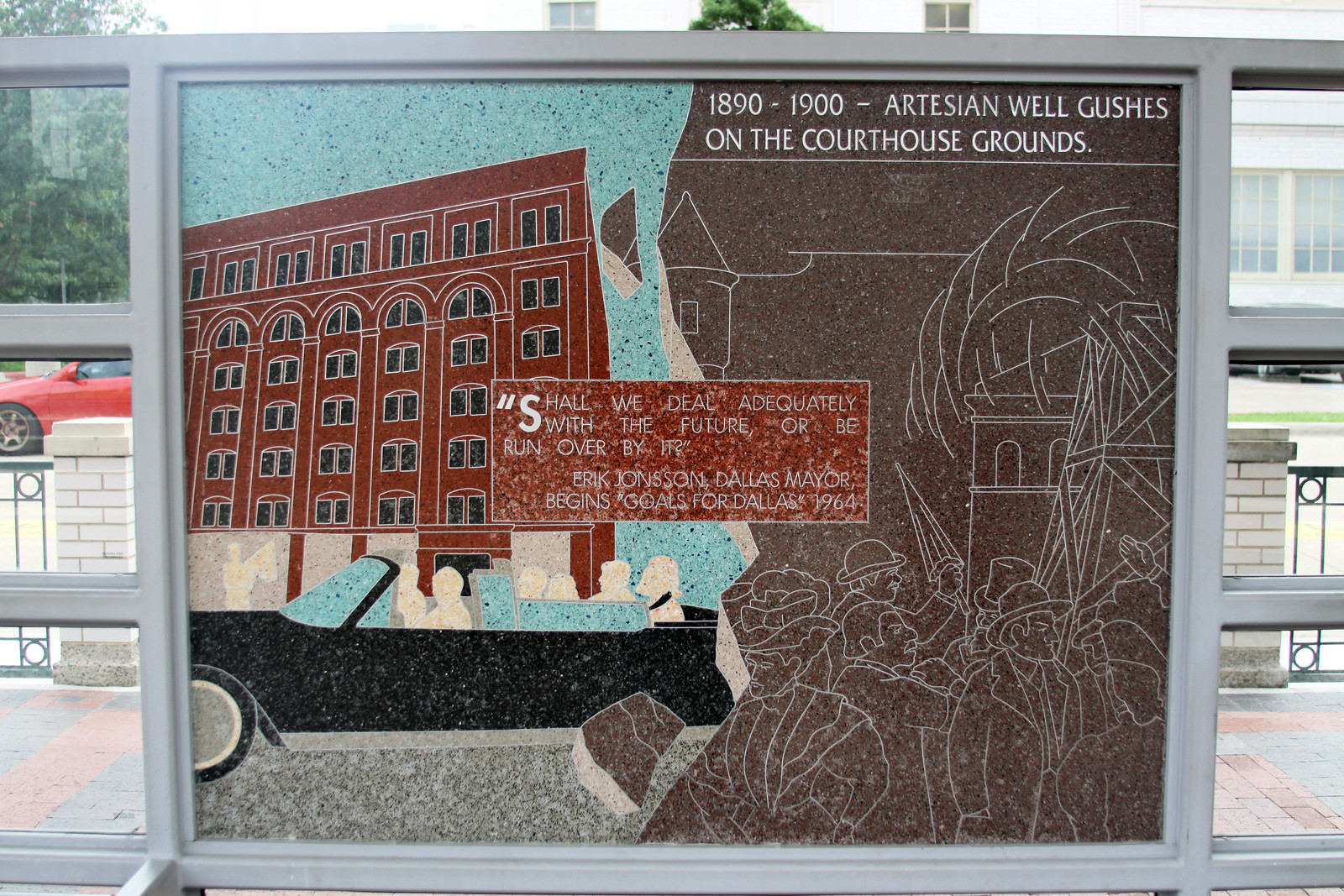The image depicts a large, detailed sign or mural, seemingly behind glass, with a gray frame encompassing it. The left half of the mural illustrates a tall, brownish-red building with numerous black windows alongside a black car driving beneath it, filled with six solid white silhouettes of people. Centered within the left side is a bold statement on a dark red background with white text that reads, "Shall we deal adequately with the future or be run over by it? Eric Johnson, Dallas mayor, begins goals for Dallas 1964." Transitioning to the right half, the background shifts to slate-colored, resembling a chalkboard with white chalk drawings of a crowd at the bottom—one person distinctly holding an umbrella—standing before several taller buildings. At the top right, in white font, the mural states, "1890 to 1900, Artesian Wells gushes on the courthouse grounds." The setting behind the mural hints at an outdoor environment with a light sky, a green tree in the left corner, and a few buildings in the distance. The entire scene evokes a historical and urban narrative, interwoven with contemplative and future-focused sentiments.